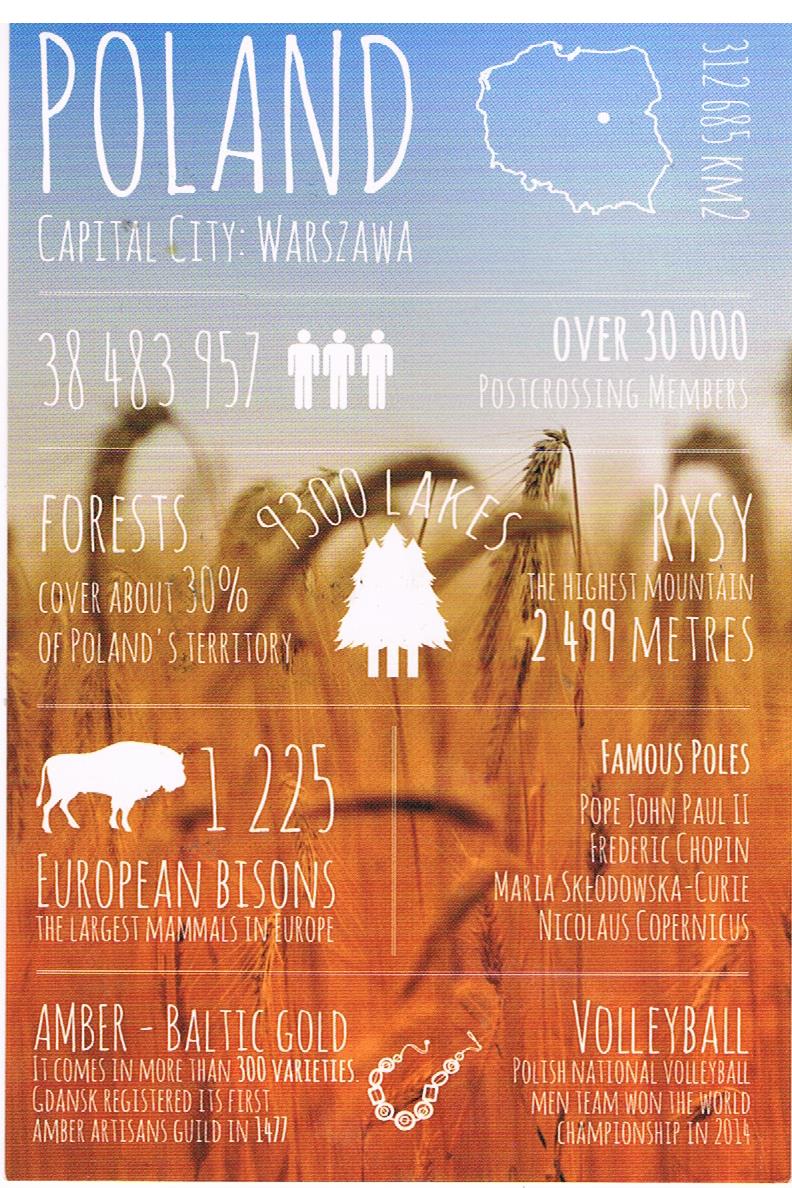The image is a poster of approximately 8 by 10 dimensions featuring an informative design about Poland against a scenic background of a wheat field transitioning from an orange hue at the bottom to lighter browns and a clear blue sky above. Overlaying this natural backdrop, the white text and icons provide various facts about Poland. At the top left, it reads "Poland, capital city, Warsaw," accompanied by an outline of the country. The text includes specific data, such as the area of Poland—312,685 km²—and its population of 38,483,957, illustrated by three stick figure men. It also highlights over 30,000 Postcrossing members.

Additional information details the country's natural resources, stating that forests cover about 30% of Poland's territory and the country boasts 9,300 lakes, symbolized by a tree icon. The poster also notes Rysy as the highest mountain at 2,499 meters and mentions the presence of 1,225 European bisons, the largest mammals in Europe. Prominent Polish figures listed include Pope John Paul II, Frederick Chopin, Maria Skłodowska-Curie, and Nicolaus Copernicus. The poster also highlights amber, known as Baltic gold, pointing out that Gdansk registered its first amber artisans guild in 1477, with amber coming in more than 300 varieties. Lastly, it references Polish volleyball, noting that the Polish National Volleyball Men's Team won the World Championship in 2014.